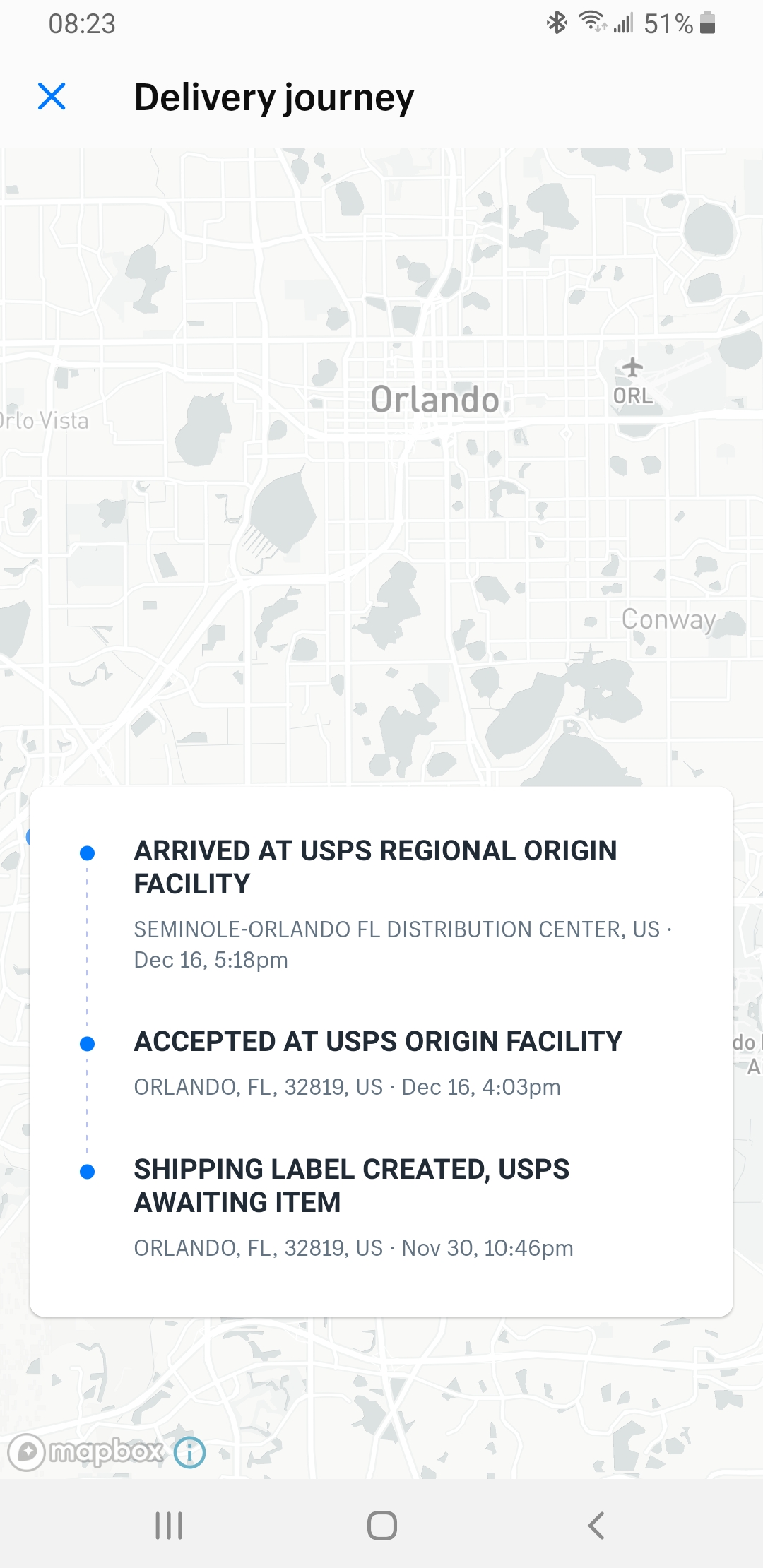A detailed screenshot of a smartphone displaying a shipping update page. At the top, the number 823 and an "X" are prominently visible, followed by the heading "Delivery Journey." The central portion of the screen features a map with a light gray background and darker gray markings, mostly rounded, indicating various locations. "Orlando" is labeled prominently in the upper center of the map, with "Vista" towards the left and "Conway" to the right.

Superimposed on this map is a white rectangle containing three blue dot indicators, each accompanied by textual details. The first blue dot reads: "Arrived at USPS Regional Origin Facility, Seminole, Orlando, Florida Distribution Center, U.S., December 16th, 5:18 AM." The second blue dot states: "Accepted at USPS Origin Facility, Orlando, Florida, 32819 U.S., December 16th, 4:03 PM." The third blue dot indicates: "Shipping Label Created, USPS Awaiting Item, Orlando, Florida, 32819 U.S., November 30th, 10:46 PM."

In the lower-left corner, the logo "Mapbox" is visible. At the bottom of the screen, a navigation bar featuring several icons allows the user to move from this page to other sections of the app.